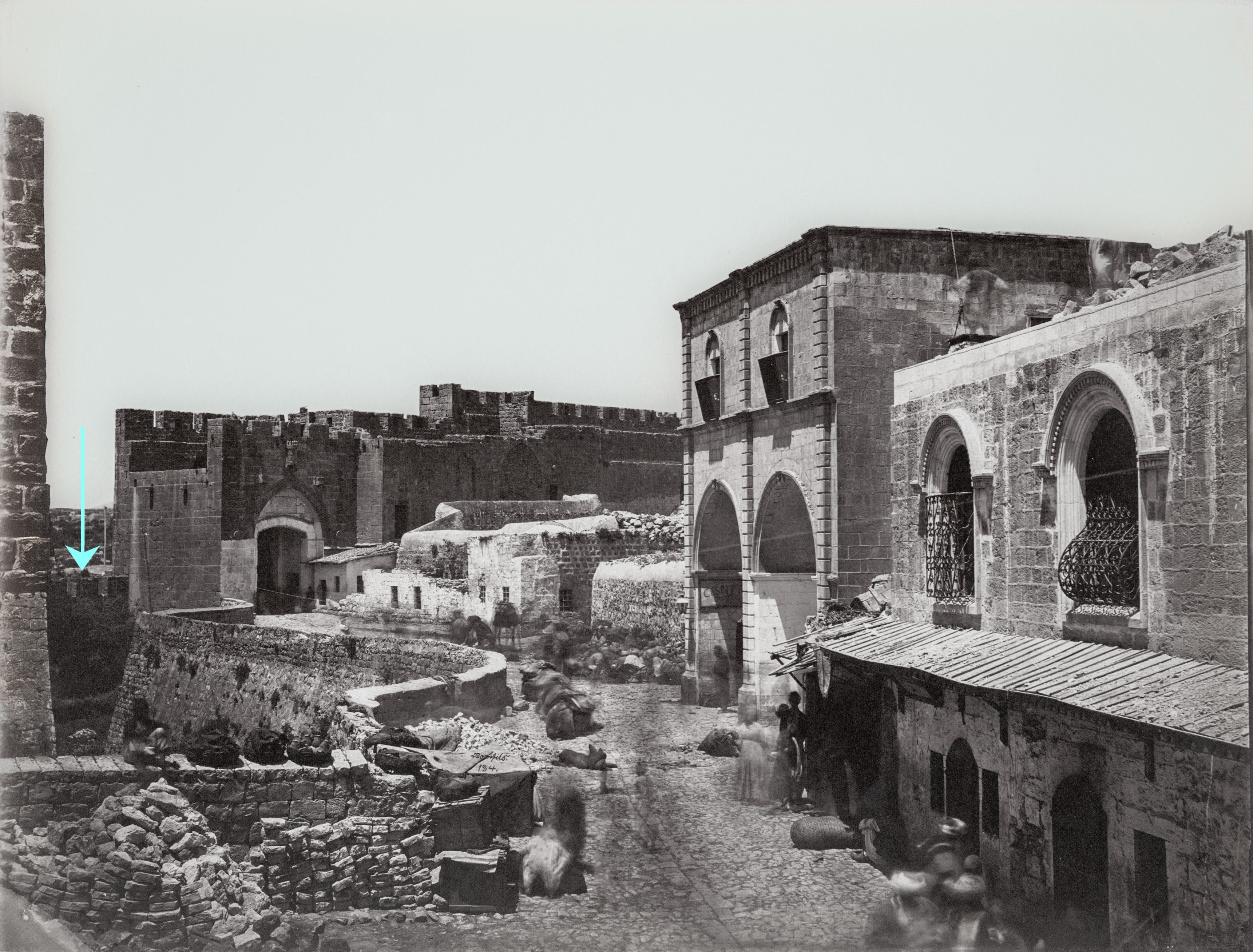This black and white photograph captures an old-looking, likely foreign town characterized by its ancient architecture. The scene features a mostly deserted street with a few people scattered around, contributing to its somewhat eerie, ghostly atmosphere. The town is fortified with a prominent walled fort, constructed from large stones and bricks, indicating its historical significance. The fort walls protect a mixture of crumbling, ancient buildings and slightly more modern structures dating back to the 1930s or 1940s, adorned with wrought iron balconies. The ground appears dusty, and an arrow in the distance seems to point towards an indistinct object, adding a sense of mystery to the image. Some blurred figures in the background enhance the image's sense of age and decay, as they appear almost ghostly, further emphasizing the town's long-standing history.